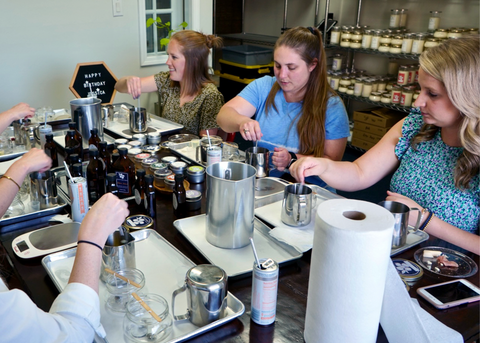This indoor photograph captures a group of six Caucasian women engaged in an activity at a large dark brown rectangular countertop or tabletop. Located in the lower right-hand corner of the image and extending diagonally towards the left, the table is adorned with various items central to their activity. The women, appearing to be in their 20s, have darker brown hair, except for one with lighter brown hair, and are dressed in floral-patterned and solid blue shirts, one notably with a flowery pattern and another in solid blue.

On the right-hand side, three women are fully visible, each stirring contents in small stainless steel pitchers with handles. On the left-hand side, we only see three sets of forearms and hands, suggesting the presence of three more women similarly engaged. Various objects are scattered across the table, including a roll of white paper towels, several dark brown to amber glass jars with black caps, and a couple of clear glasses. A silver tray with white paper, likely used for their crafting materials, is also visible.

In front of these women are small jars that could contain oils, possibly for making soaps, perfumes, or essential oils, though the exact nature of their project is unclear. Some women have beverages with straws next to their trays, and there are plates near their stations. A black hexagon-shaped sign with a wooden frame and white text sits on the table, reading "Happy Birthday," adding a celebratory context to the scene.

The backdrop features a light gray wall on the left and metal shelving units on the right, holding small jars with light yellow labels, brown cardboard boxes, and a mix of containers. A glimpse of a window with a white frame and a green leafy plant on the sill further decorates the area.